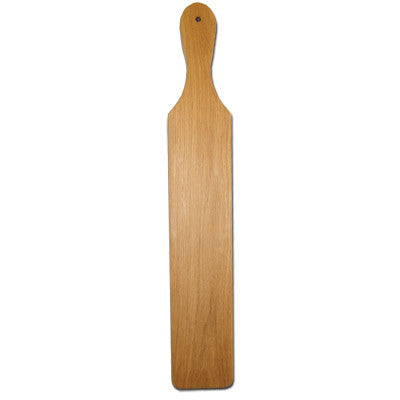The image depicts a single, long wooden object that appears to be either a serving board or a paddle, set against a plain white background. The object is oriented vertically and showcases a handle shaped like a teardrop with a small hole at the end, presumably for hanging, though no string is present. The handle gradually widens into a rectangular body. The wood exhibits a medium tannish color with the grain running vertically. The central portion of the board is lighter, whereas the handle and end have slightly darker wood grain, adding a subtle contrast. The surface appears new and clean, with a noticeable gloss highlighted by a light source that creates a shiny effect on the wood. The utensil is estimated to be over a foot in length and is resting against the white background, providing a clear and unobstructed view of its structure and finish.